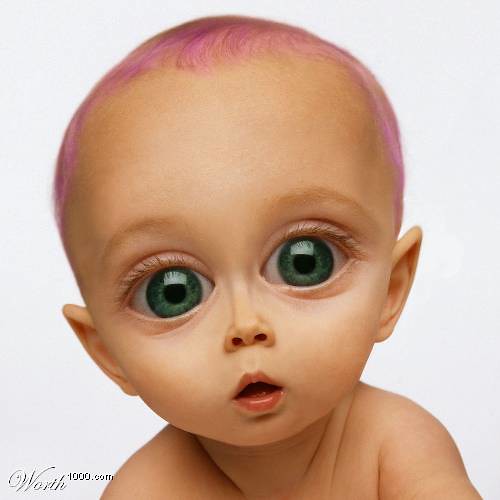The image depicts a distorted portrait of an infant from the shoulders up, set against a plain white backdrop. The baby's head appears unusually large, resembling an alien-like figure, with features exaggerated to an eerie degree. The infant has sparse, pink-hued hair, oversized eyes that are either blue or green, and small, pointed ears that give an elfin impression. The tiny nose and mouth further contribute to the bizarre alteration of the original photograph. The lower left-hand corner of the image bears a logo that reads "WORTH1000.com." Overall, the picture evokes a sense of unease, reminiscent of grey alien imagery.